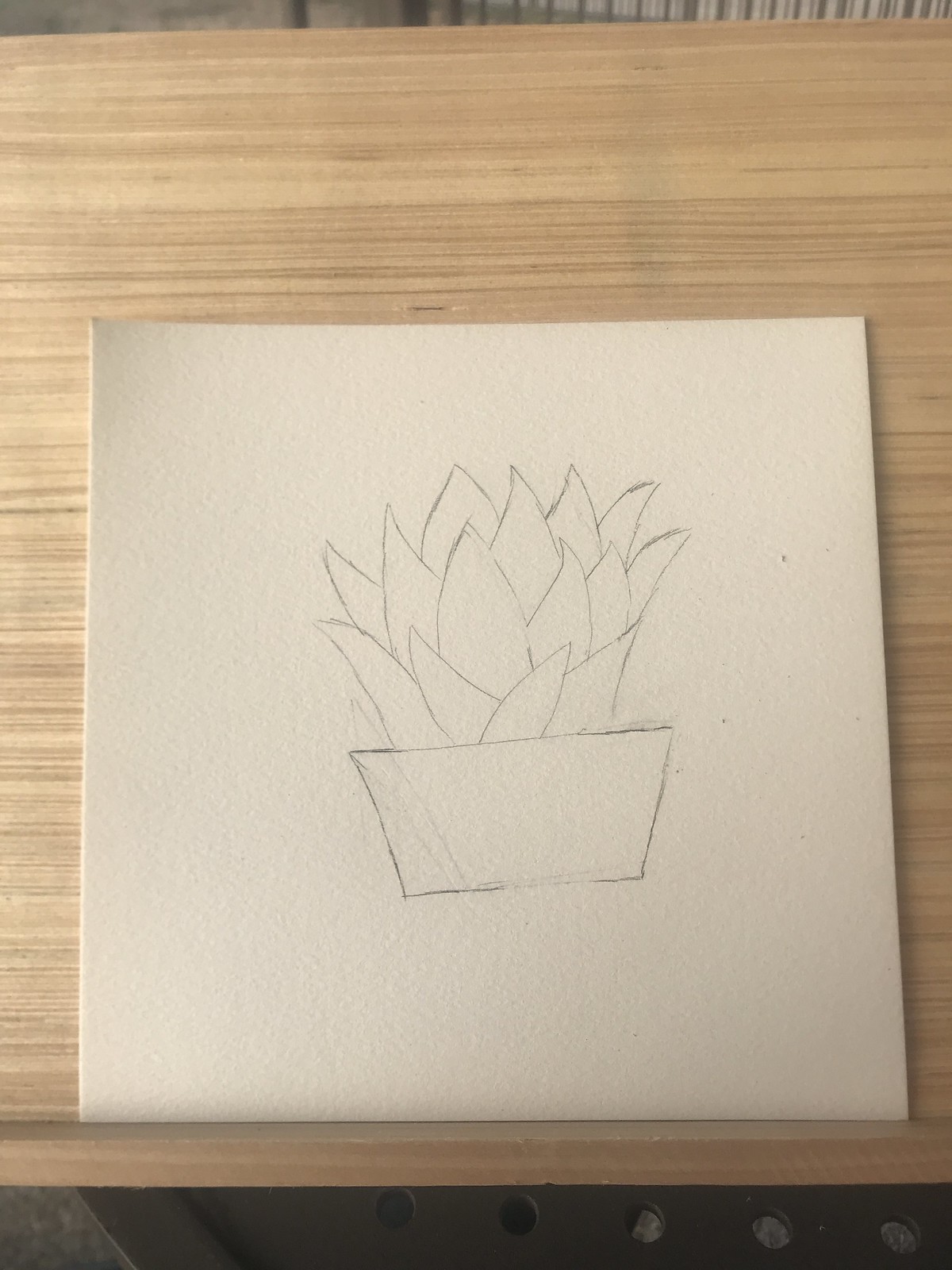The image showcases a detailed pencil drawing of a plant, possibly a succulent with many spiky leaves, housed in a rectangular, flared pot. The drawing is centered on an off-white, square piece of paper, which has slight creases and resembles watercolor paper. This paper is laid on a light brown wooden table with visible darker striations. Towards the left of the image, a metal chair can be seen tucked under the table. The table itself occupies most of the image, extending from the top left to the top right. The background shifts from a lighter gray with spots in the left corner to a uniform dark gray with five holes on the right, showing a mix of black and light gray behind them. A small section at the very top of the image reveals a beige-colored fabric, possibly a curtain with slight folds. The overall setting suggests the scene is indoors, perhaps in a home or a classroom.